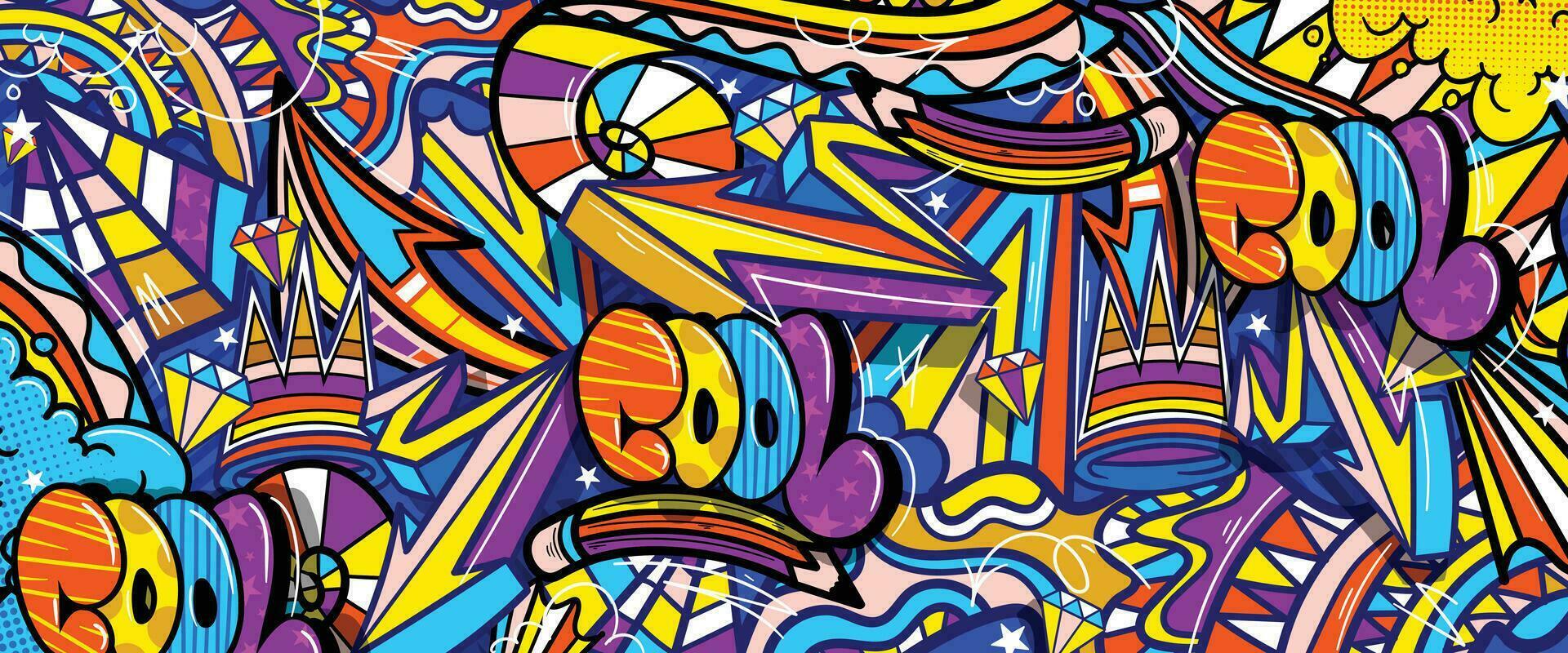This vibrant, abstract, and colorful graphic design features a retro, cartoon-like aesthetic reminiscent of 80s hip-hop graffiti. The composition is a medley of diverse shapes, such as crowns, arrows, pennants, pyramids, pencils, and diamond shapes, all intricately intertwined. The design is dominated by a palette of purples, yellows, turquoise, blues, reds, white, light blue, and brownish orange. Notably, the word "cool" appears three times in different colored letters: starting in the bottom left-hand corner, then repeated in the middle, and finally in the upper right-hand corner. Each instance of the word showcases a unique color pattern—the red 'C' with yellow lines, the yellow first 'O' with orangish polka dots, the light blue second 'O' with dark blue lines, and the purple 'L' with lighter purple stars. Triangular shapes, swirls, clouds, and arrows add to the lively, dynamic feel of the piece, making it reminiscent of colorful wrapping paper. The meticulous layering of elements gives the image depth and dimension, making it appear as a vivid collage bustling with animated, digital artistry.